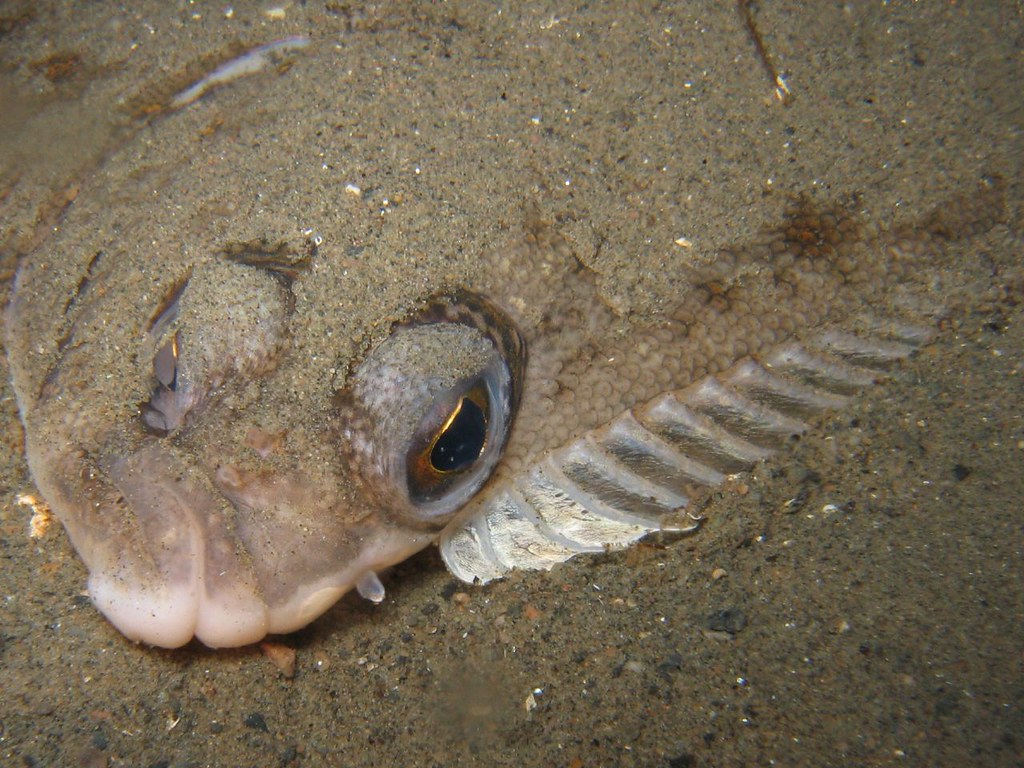The image is a detailed, close-up photograph of a bottom-dwelling fish partially buried in the sandy and rocky seafloor. The fish, positioned from the top right corner to the middle left, exhibits a range of colors including tan, white, orange-brown, black, and gray. Its flat, thin body is largely covered in sand, with visible fins on the left side. The fish's skin has a beige-brown hue with brown spots, and its big, expressive eyes feature a golden outer edge and a dark iris, possibly with a blue border. The fish seems camouflaged against its surroundings, which consist mainly of light brown sand interspersed with small black rocks. The marine setting emphasizes the fish's ability to blend into the underwater environment, highlighting details such as its reflective, metallic-like skin and whitish mouth.